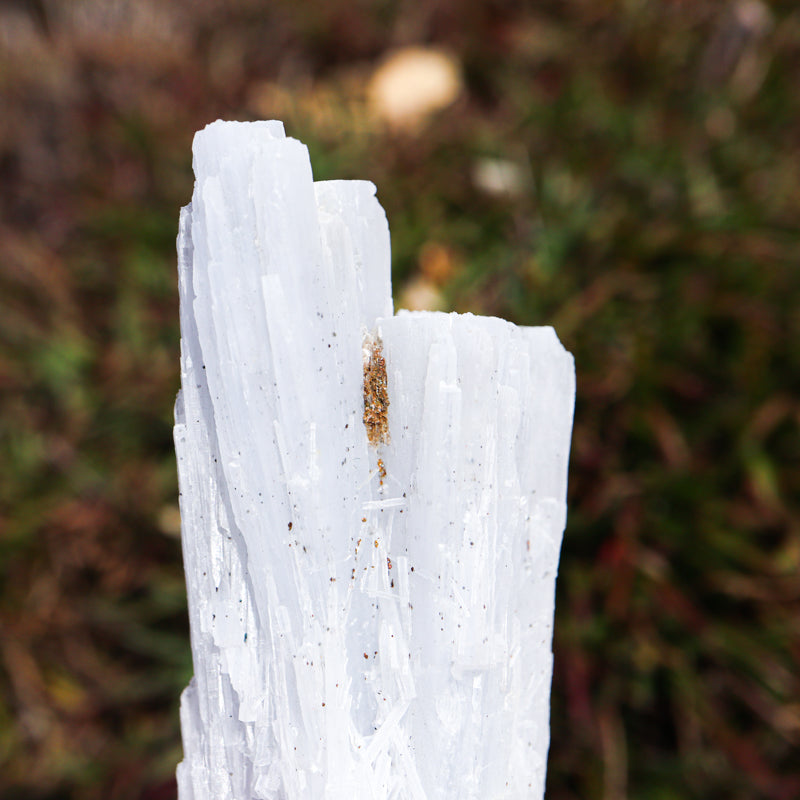In this detailed image, the central focus is on three distinct, white crystalline structures, reminiscent of sugarcane, stone, or rock. Positioned in the heart of the image, these structures resemble a massive statue-like crystal, their pristine whiteness almost as radiant as fresh snow, with an apparent crystalline texture. The three stalks vary in height, creating a multi-level formation with a noticeable crevice where the crystals have split.

Intricately detailed, the surface of these crystals is peppered with tiny specks of orange-brown dust and possible small bugs, most densely concentrated towards the top of the structure. Black dots, potentially spider eggs or hatching bugs, are scattered across the surface, adding to the intricate detail.

The background of the image is artistically blurred, suggesting an outdoor setting. Shades of green and brown, along with indistinct purple leaves, hint at a forest floor adorned with shrubbery and foliage, creating a natural, earthy backdrop that contrasts with the stark whiteness of the central crystalline structures.